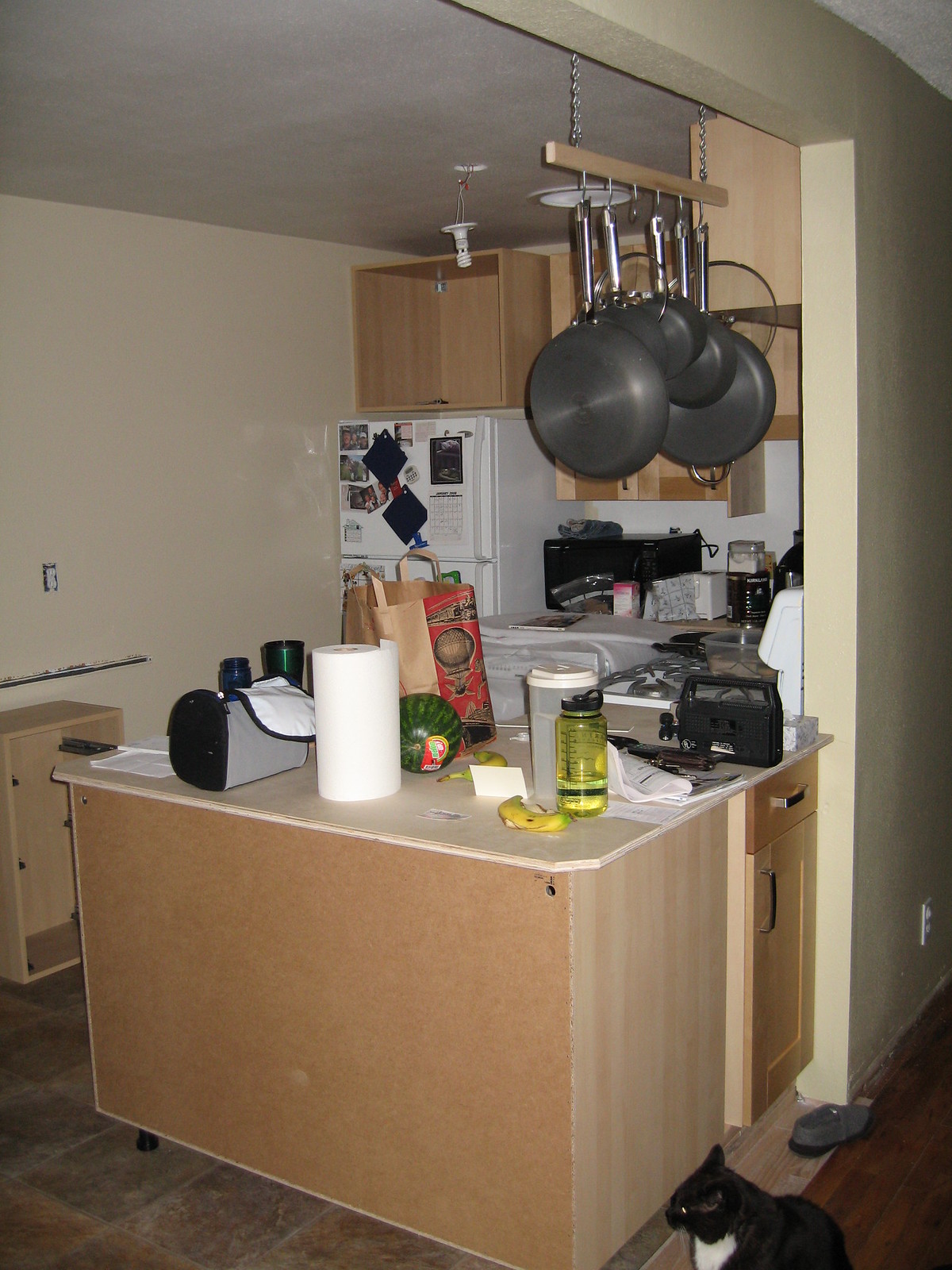In this photo, a cat is lounging on the floor amidst the clutter of a very messy kitchen. The kitchen is C-shaped with light wood veneer cabinetry. On the left side towards the back, there's a white refrigerator. Adjacent to it, a short counter holds a black microwave. Above, a hanging wooden shelf supports several plants. Scattered across the kitchen, there's a chaotic assortment of items: a grocery bag with a watermelon next to it, a yellow water bottle, cups, a banana, and possibly a CD player on the nearest counter. A lone shoe also lies on the floor. The overall impression is of a cramped and cluttered apartment kitchen.